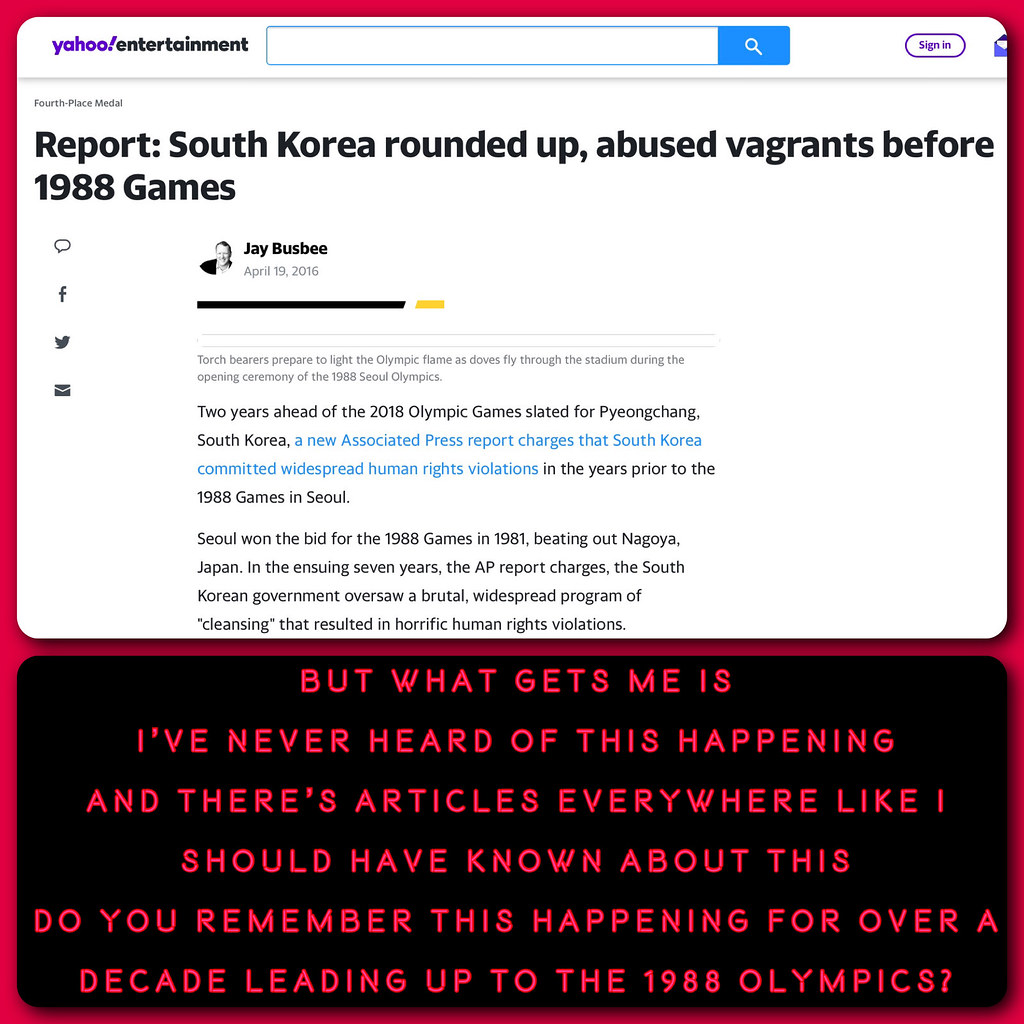The image depicts a screenshot from Yahoo Entertainment featuring a detailed news snippet. At the very top left corner, "Yahoo Entertainment" is prominently displayed alongside a search bar and an email sign-in icon symbolized by a mail symbol. Below this, the article headline reads, "Report South Korea Rounded Up Abused Vagrants Before 1988 Games," followed by the author's name with a small thumbnail photo next to social sharing icons including chat, Facebook, Twitter, and email.

The article discusses an Associated Press report alleging that South Korea committed severe human rights violations in the years leading up to the 1988 Seoul Olympics. The report claims that after winning the bid in 1981, the South Korean government engaged in a brutal "cleansing" campaign that resulted in widespread abuse. The story cuts off after several detailed paragraphs detailing these accusations.

The entire news snippet is outlined in a bright red border. Below this section, there is a distinct black rectangle also highlighted with a red border. This section contains a quote in bright pink text expressing surprise and disbelief at the reported events, stating, "But what gets me is I've never heard of this happening, and there's articles everywhere like I should have known about this. I remember this happening for over a decade leading up to the 1988 Olympics." This comment suggests a personal reflection on the article's revelations, adding a layer of reader engagement and skepticism.